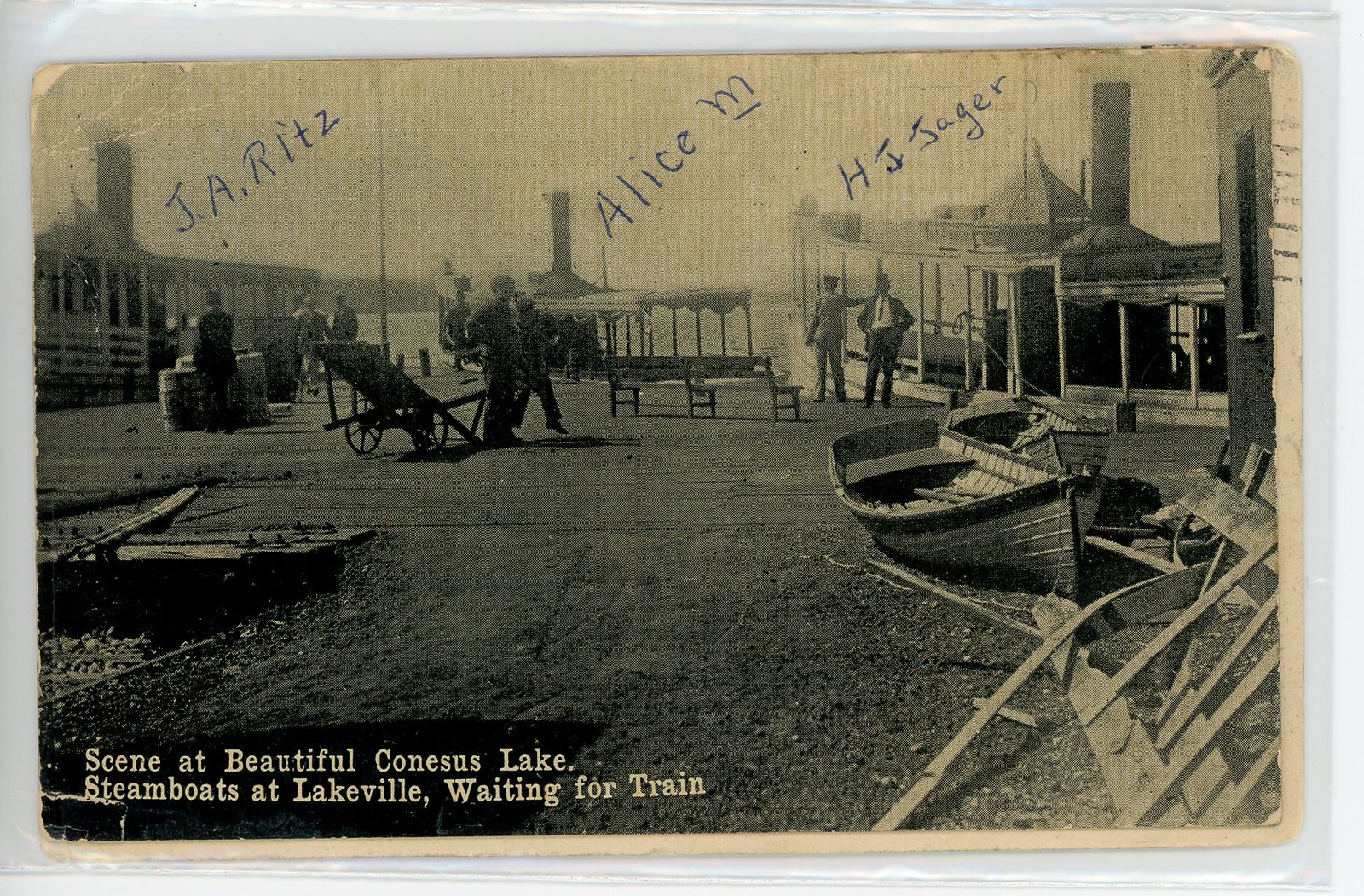In this old black-and-white photograph, encased in a protective plastic sleeve, we see a bustling waterfront scene that appears to be a beach or pier at Conesus Lake. The scene showcases three steamboats: one on the left labeled "J.R. Ritz," one in the center marked "Alice M.," and one on the right identified as "H.J. Yeager," with these names hand-written in blue ink above each vessel. 

The image captures a variety of details. In the foreground, two rowboats rest on the ground amidst pieces of wood, possibly part of a shipyard setting. Several men are standing around, one of whom is distinctly wearing a suit, tie, and hat near the steamboat labeled "H.J. Yeager." To the right, higher up in the scene, there are buildings with open sides but roofs intact, giving the area a somewhat busy yet not overly crowded appearance. You also can spot a smokestack in the center distance, though it’s unclear whether it belongs to another steamboat or a chimney due to the blurriness of the aged photo.

The photo’s captions include a handwritten inscription at the bottom left, albeit in a slightly faded tan color, reading: "Seen at Beautiful Conesus Lake, Steamboats at Lakeville Waiting for Train." The rectangular photograph with rounded edges shows signs of aging, with little wrinkles and tears, adding to its historical charm.